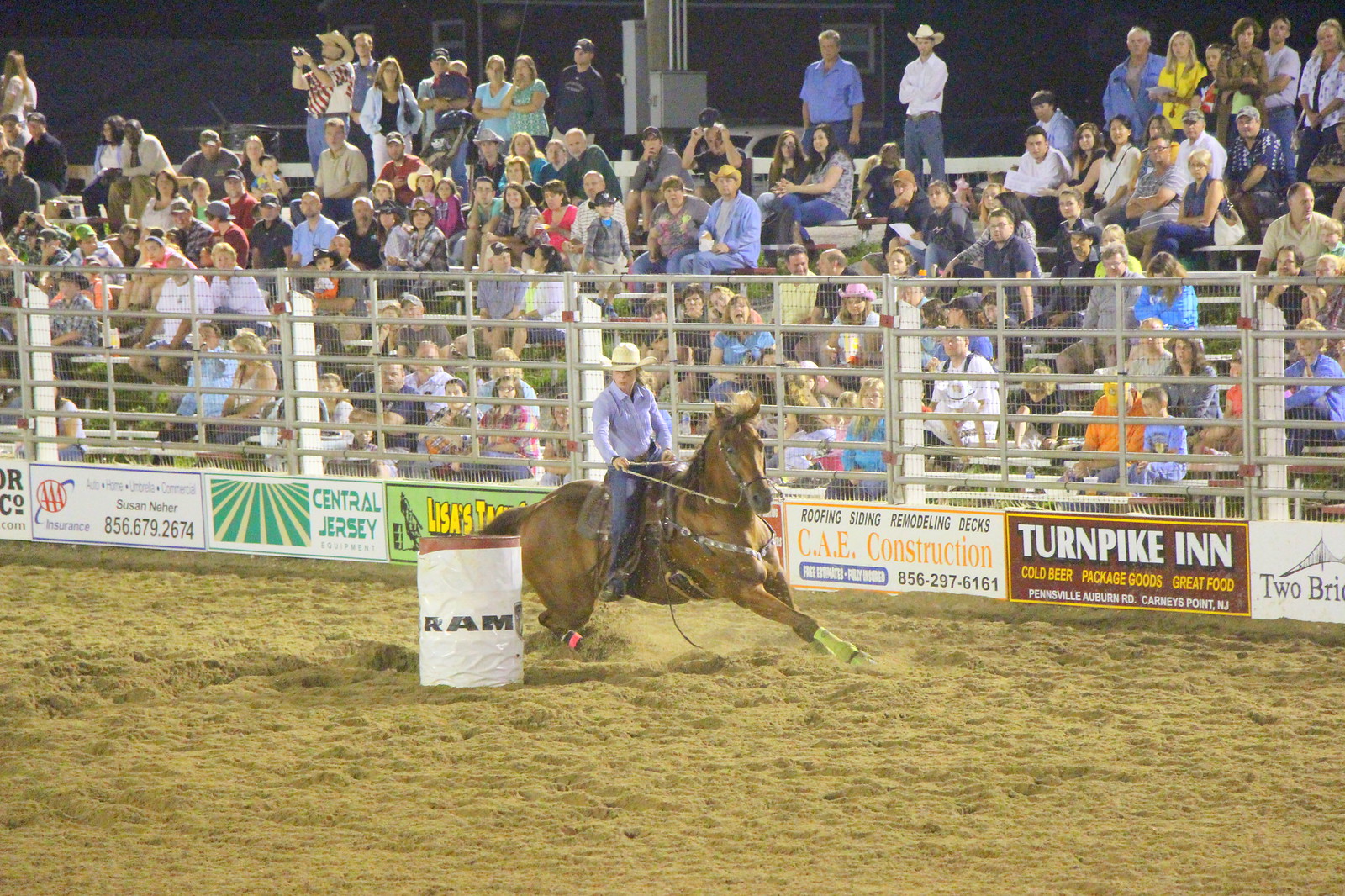This horizontally-oriented photograph captures a vibrant rodeo scene at night inside a stadium. In the foreground, a light brown horse, with harnesses and a saddle, is in mid-stride as it skillfully navigates around a cylindrical barrel marked with "RAM." The rider, clad in a light blue shirt, blue jeans, and a white cowboy hat, holds the reins in his right hand, guiding the horse in a sharp right turn around the barrel. The horse's front legs are stretched forward, while its back legs are tucked in, kicking up white dirt from the arena floor. Surrounding the arena is a tall fence adorned with advertising banners for various companies, such as Turnpike Inn, CAE Construction, and Central Jersey. Behind the fence, a large crowd of spectators, many dressed in casual clothes that include blue jeans and cowboy hats, fills the bleachers. The stadium’s roof, supported by posts, can be seen in the background, as well as the dark gray sky, which adds a dramatic backdrop to the event. The photograph captures the dynamic energy and excitement of the moment, with the rider and horse in perfect unison as they compete in this thrilling rodeo contest.